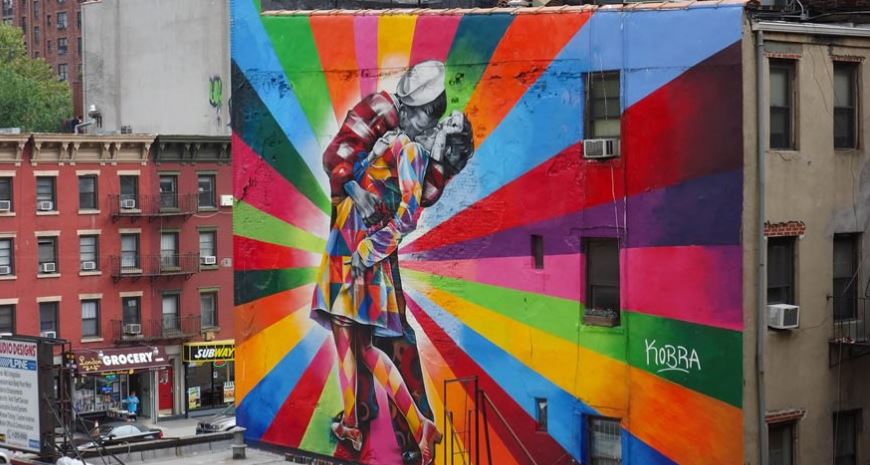On the side of a large urban brownstone building in New York City, there is a vibrant graffiti mural that spans the entire wall. The mural features a dynamic background showcasing every color of the rainbow in a gradually fanned out kaleidoscope pattern. Prominent colors include green, orange, yellow, pink, salmon, various shades of blue, and violet. At the center of the mural, there is a graffiti reproduction of the iconic photograph from World War II, where a sailor passionately kisses a woman, bending her backwards in a dramatic embrace. This central image is infused with the same rainbow colors as the background, giving it a prism-like effect rather than the original black and white. To the far right of the mural, in white lettering, is the word "Kobra," likely the artist's signature. The mural is set against a backdrop of typical New York style urban scenery, with multi-story brick apartment buildings above bodegas and small shops on the ground floor. Air conditioning units jut out from the windows of these buildings, further grounding the mural in its urban context. The scene is illuminated by the natural light of a cloudy day, enhancing the mural's vibrant and dynamic visual impact.